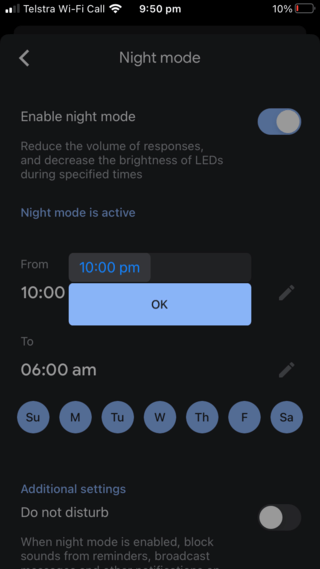The image showcases a phone screen with a black background. In the upper left corner, the status bar displays "Telstra Wi-Fi call" alongside a Wi-Fi signal icon. The time is shown in the middle as "9:50 p.m.," while the battery icon on the upper right indicates 10% remaining battery life.

Below the status bar, there is a left-facing arrow next to the label "Night Mode." Directly beneath this, the phrase "Enable Night Mode" appears, with a switch on the right set to "on." The next line reads, "Reduce the volume of responses," followed by "Decrease the brightness of LEDs during specified times."

Further down, a blue-highlighted text states "Night Mode is active." Below this, it specifies that the mode is set from "10:00 p.m." (in blue text) to "6:00 a.m." (in white text), with editable times indicated by small pencil icons. Days of the week are represented by blue circles, and additional settings are listed under "Do Not Disturb" in a yellowish color.

When Night Mode is enabled, it blocks sounds from Reminders and Broadcasts, highlighted by a gray circle.